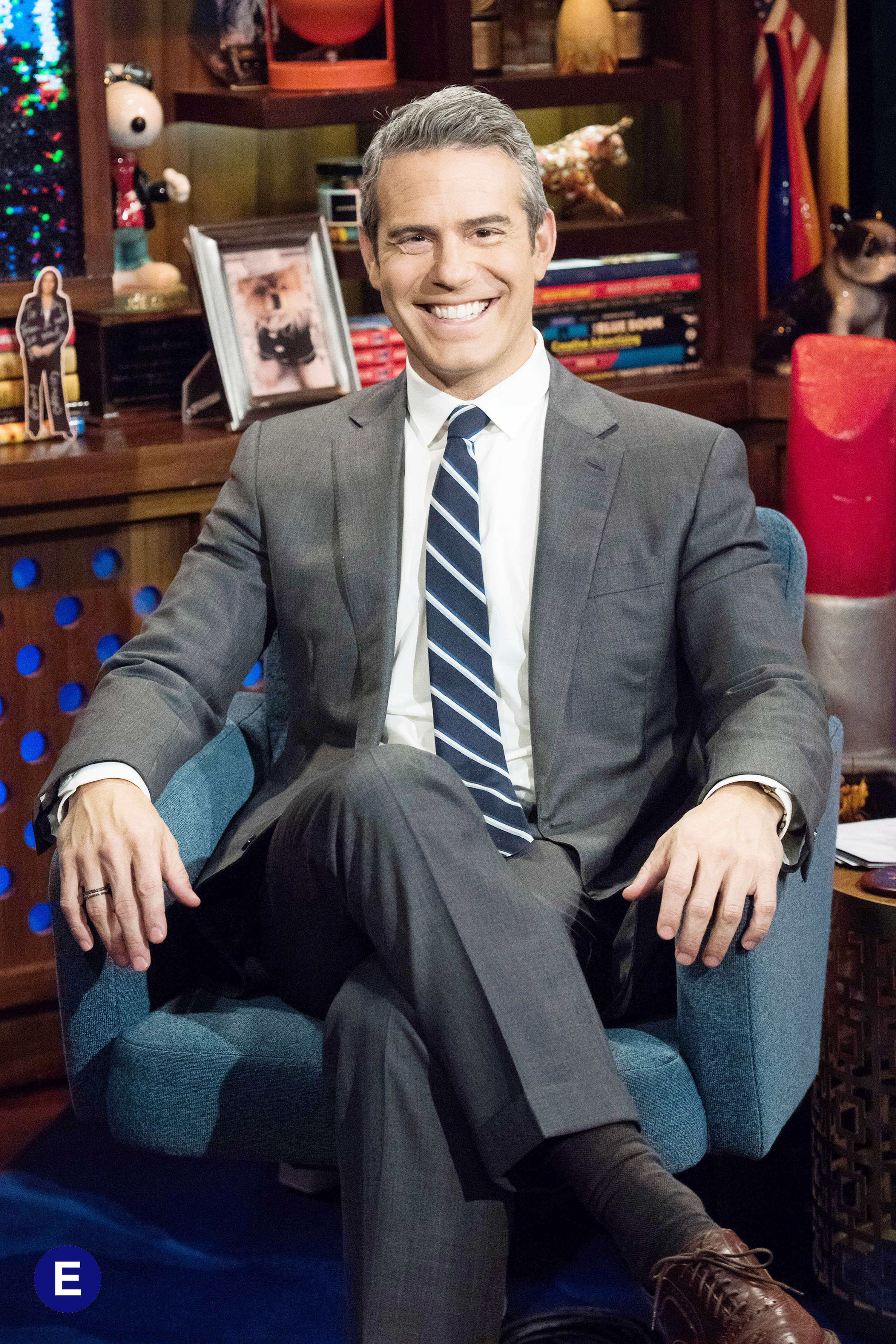In this image, a man is seated in a cushy blue chair with armrests, radiating a warm, big smile that showcases his white teeth. He has short, slicked-back, salt-and-pepper hair and is dressed sharply in a gray suit paired with a white shirt and a blue and white striped tie. His attire is complemented by shiny brown shoes and a wedding ring on his ring finger. Behind him, the office setting features a variety of objects, including wooden cabinets, bookshelves with frames, books, and playful items such as a Snoopy figurine and dog or cat statues. An American flag is visible in the corner, and the office space includes blue carpeting and a brown desk adorned with blue cutout circles and various colorful decorations. The man, likely Andy Cohen, is set against this eclectic office background, adding a whimsical touch to the professional atmosphere.